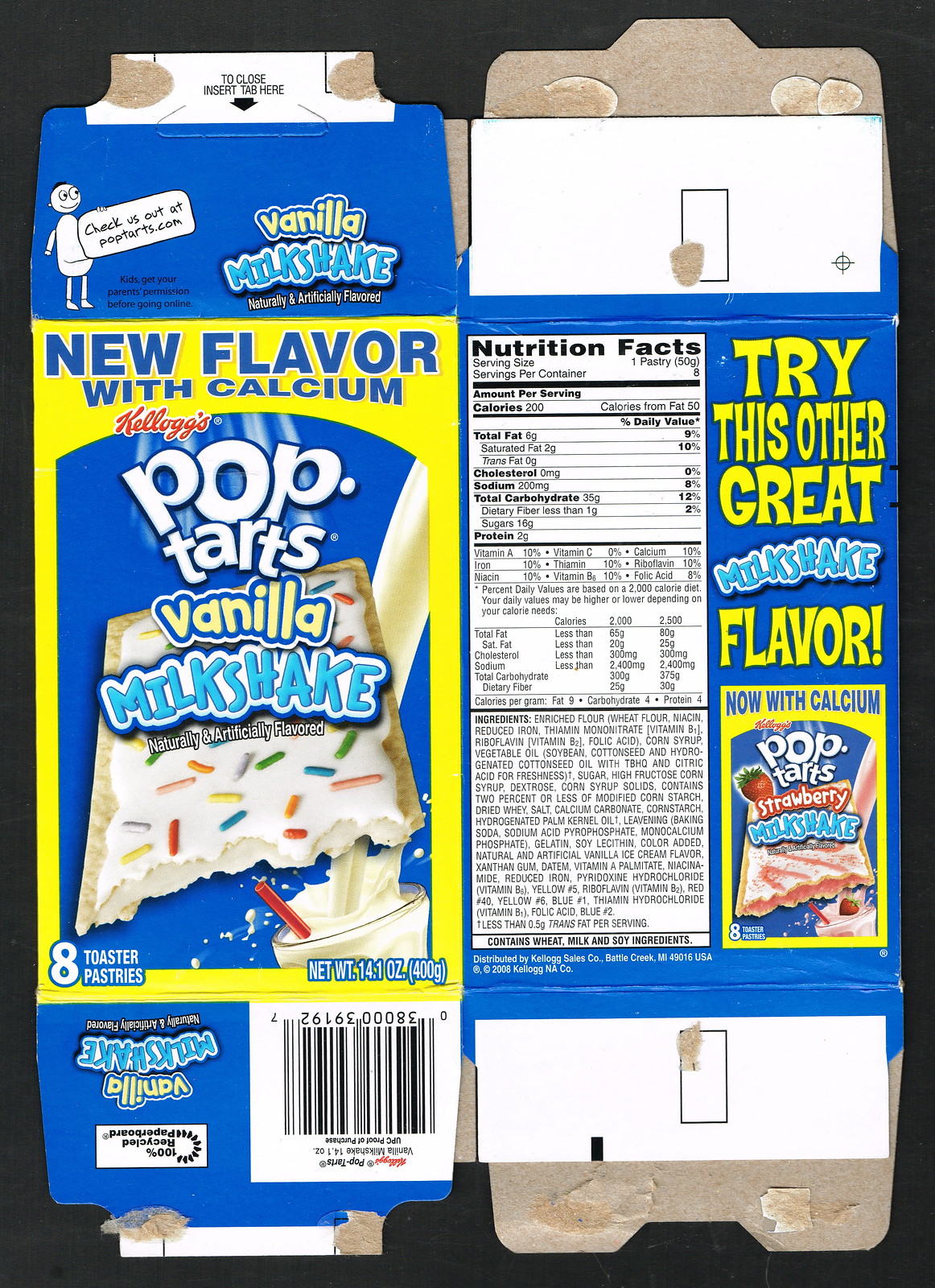This detailed photograph depicts a thoroughly flattened box of Kellogg's Pop-Tarts in a vanilla milkshake flavor. At the top of the box, there's an image of a person with text encouraging viewers to visit "pop-tarts.com." Below this, bold lettering announces the "Vanilla Milkshake" flavor. A vibrant yellow banner with blue text highlights that this is a "New Flavor with Calcium." 

The centerpiece of the box features an enticing image of a Pop-Tart, adorned with white icing and colorful sprinkles. To its right, an image shows milk cascading down from the top right into a transparent glass, which contains a red straw, emphasizing the milkshake theme. 

Toward the bottom, a barcode is prominently displayed. On the left side, the package notes that it contains "8 Toaster Pastries." 

The right side (the back of the box) provides detailed nutritional information and a list of ingredients. Additionally, in a bright yellow font, there's a suggestion to try another flavor, specifically "Strawberry Milkshake," accompanied by a visual of the strawberry version of the product.